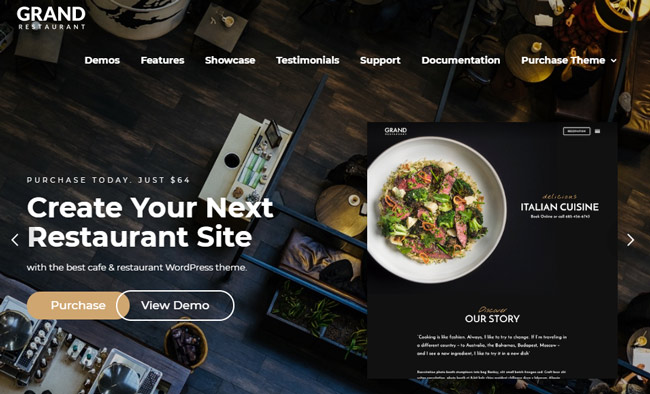In the top left corner of the website, bold white capital letters spell out "GRAND." Just below, "RESTAURANT" is written, with the "S" and "T" highlighted in a slanted gray square, adding a subtle visual distinction. The rest of the letters in "RESTAURANT" are spaced out evenly to match the width of the "GRAND" above. 

To the right of this title, the main menu begins, featuring options in small, bold white text: "DEMOS," "FEATURES," "SHOWCASE," "TESTIMONIALS," "SUPPORT," "DOCUMENTATION," "PURCHASE THEME," each indicating further navigation options. After "PURCHASE THEME," a downward-pointing arrowhead suggests the presence of a submenu.

Below this main navigation, on the left side, the text "PURCHASE TODAY" is presented in very small white letters with notable character spacing, followed by "$64." Beneath this, in bold white text, a prominent header proclaims, "CREATE YOUR NEXT RESTAURANT SITE." Further down, a description reads, "WITH THE BEST CAFE AND RESTAURANT WORDPRESS THEME."

In the center, two overlapping ovals provide calls to action: the first oval is beige or gold-tinted with the word "PURCHASE" in white, while the second is outlined in white with a transparent background, featuring the text "VIEW DEMO."

The background is a dark wooden surface adorned with various gadgets, some of which are copper. In the bottom left, there's a metal gadget with numerous gears. On the right, you can glimpse a menu that appears to narrate the restaurant's story. In the top left corner, a white plate presents a steak salad, adding a touch of culinary focus to the design.